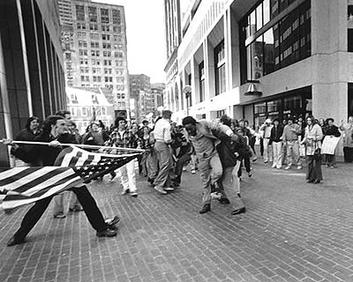In this striking black and white photo, a dramatic urban scene unfolds in what appears to be a downtown American city. The image captures a large crowd of people standing between two multi-story buildings with brick walkways underfoot, suggesting a city center plaza. In the foreground, there is a palpable tension as several individuals seem to be locked in a struggle. To the left, a man with dark hair and dark clothes holds a United States flag like a spear, gripping it with both hands and pointing it forward in a confrontational manner. He stands with his legs spread, seemingly poised to strike. To his right, two other people appear to be grabbing each other and struggling. The backdrop is lined with towering skyscrapers, one of which stands prominently in the distance, adding to the canyon-like atmosphere of the urban environment. The scene is chaotic and the nature of the confrontation suggests a possible protest, with individuals appearing to argue and engage in what may be a fistfight, although no signs are visible to confirm the exact context.